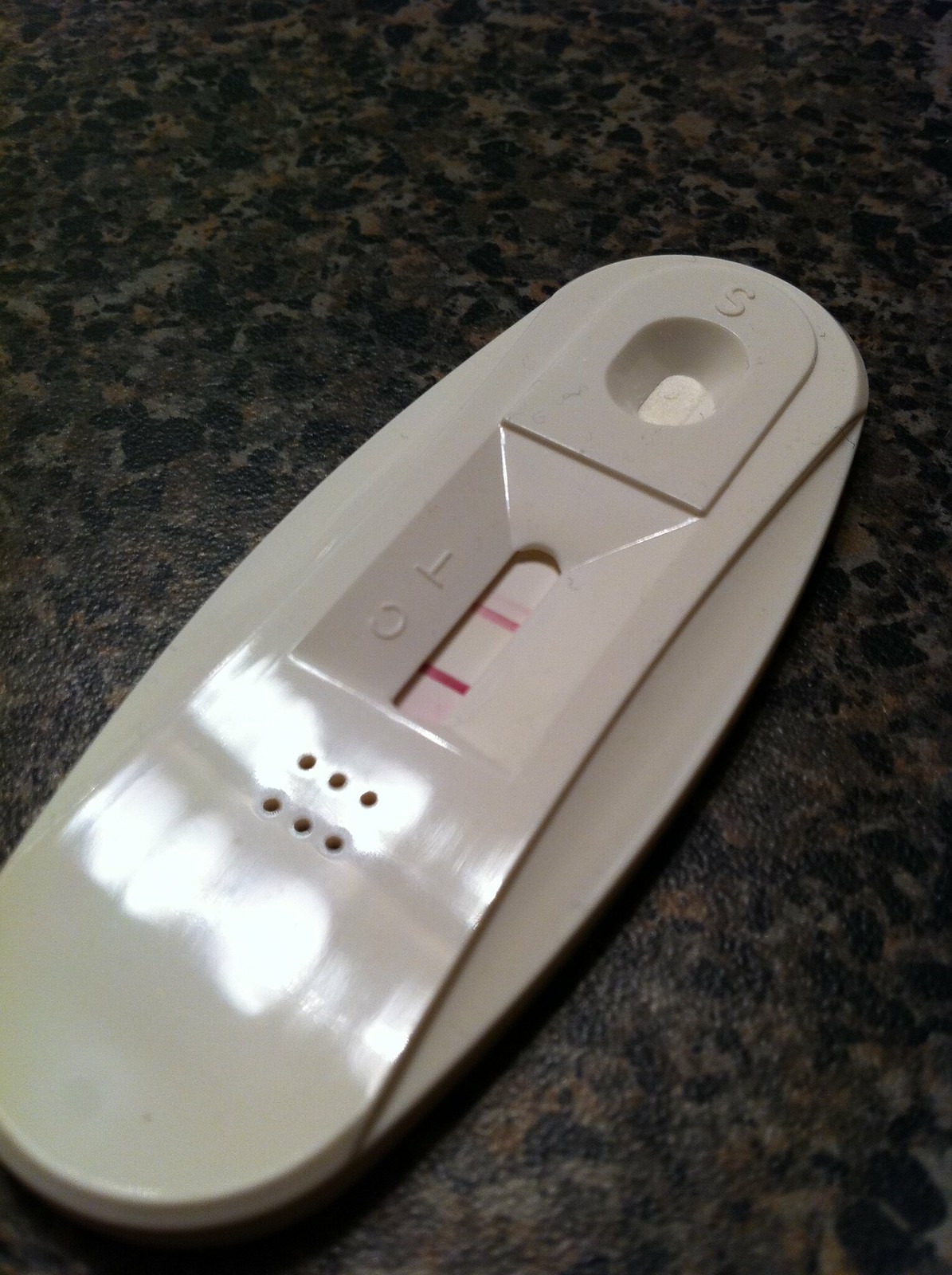The image showcases a COVID-19 test kit, specifically the test portion of the kit, placed on a vinyl countertop with a mottled pattern of gray, black, and dull brown hues. The test kit itself is made of white plastic and has an elongated oval shape with a raised section running down its middle. Reflective lights on the surface reveal its shiny texture. At the near end, there are six circular indentations arranged in two rows of three, positioned centrally. In the middle section, there is an oval window accompanied by the letters "C" and "T" on the far side, which appear upside down from the viewer's perspective. Within this window, two dark pink lines are visible—one dark line next to the "C" and a lighter line next to the "T". A third, faint line can be seen adjacent to the line next to the "T". At the far end of the test kit, there is a smaller, oval-shaped hole labeled with the letter "S".